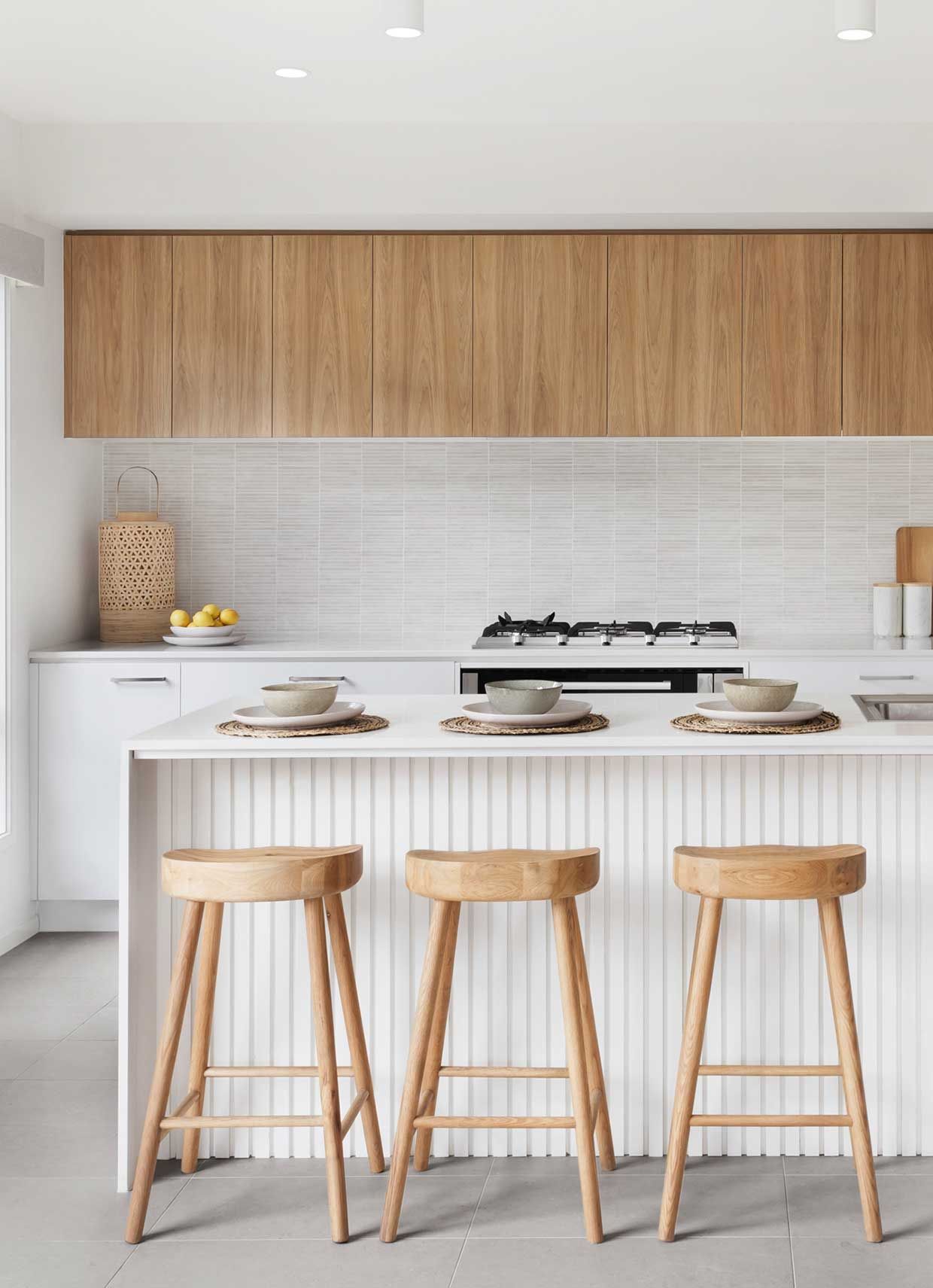This photograph captures a bright, modern kitchen with an all-white theme, illuminated by natural daylight. In the foreground, three wooden stools with round seats and no backrests are positioned in front of a pristine white kitchen island. Each stool faces a neatly arranged setting of light-colored plates and bowls on circular placemats. The countertop is spacious and uncluttered, emphasizing the minimalist design, with a bowl of lemons adding a touch of color.

Behind the island, the kitchen features sleek wooden cabinets without visible hardware, arranged in a seamless, flush design. Below them are white lower cabinets and countertops, accentuated by silver hardware and a grayish-white tile backsplash. The stovetop is integrated into the counter, which remains mostly clear except for a decorative wood vase and the mentioned bowl of lemons. The floor is composed of gray tiles, adding a subtle contrast to the otherwise white and light oak tones of the kitchen. The overall ambiance suggests a clean, organized, and airy space, epitomizing modern kitchen design.